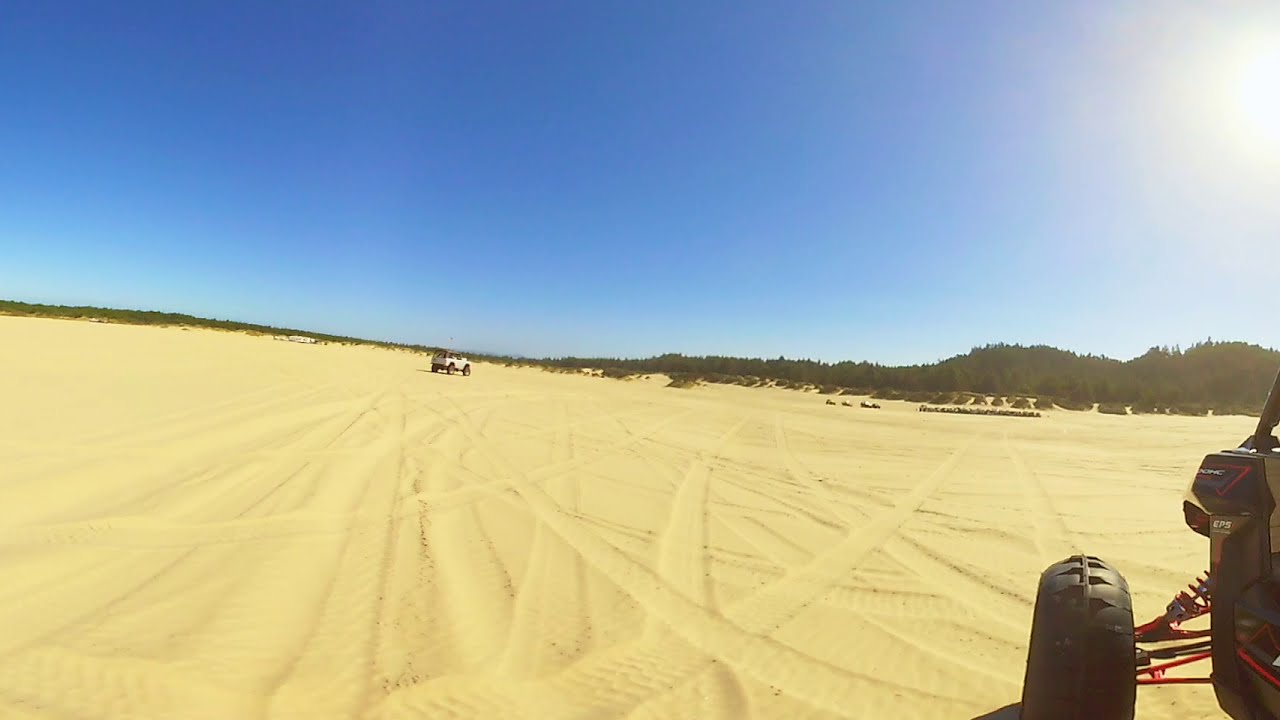The image captures a bright, sunny outdoor scene dominated by a sprawling sand dune under a clear blue sky. It's likely close to mid-morning, given the position of the bright sun up in the sky. The golden sand, which covers most of the image, is marked with numerous tire tracks crisscrossing in various directions. On the lower right side, there's a partial view of a black four-wheeler, hinting at some fun off-road activity. In the far distance, near the horizon, a small jeep or white car can be seen driving across the sand. Along the horizon line, there's a strip of trees and shrubbery that starts on the left and gradually leads to taller trees on the right. The wide, clean expanse of sand gives the place a serene, somewhat desolate feel despite the presence of vehicles.